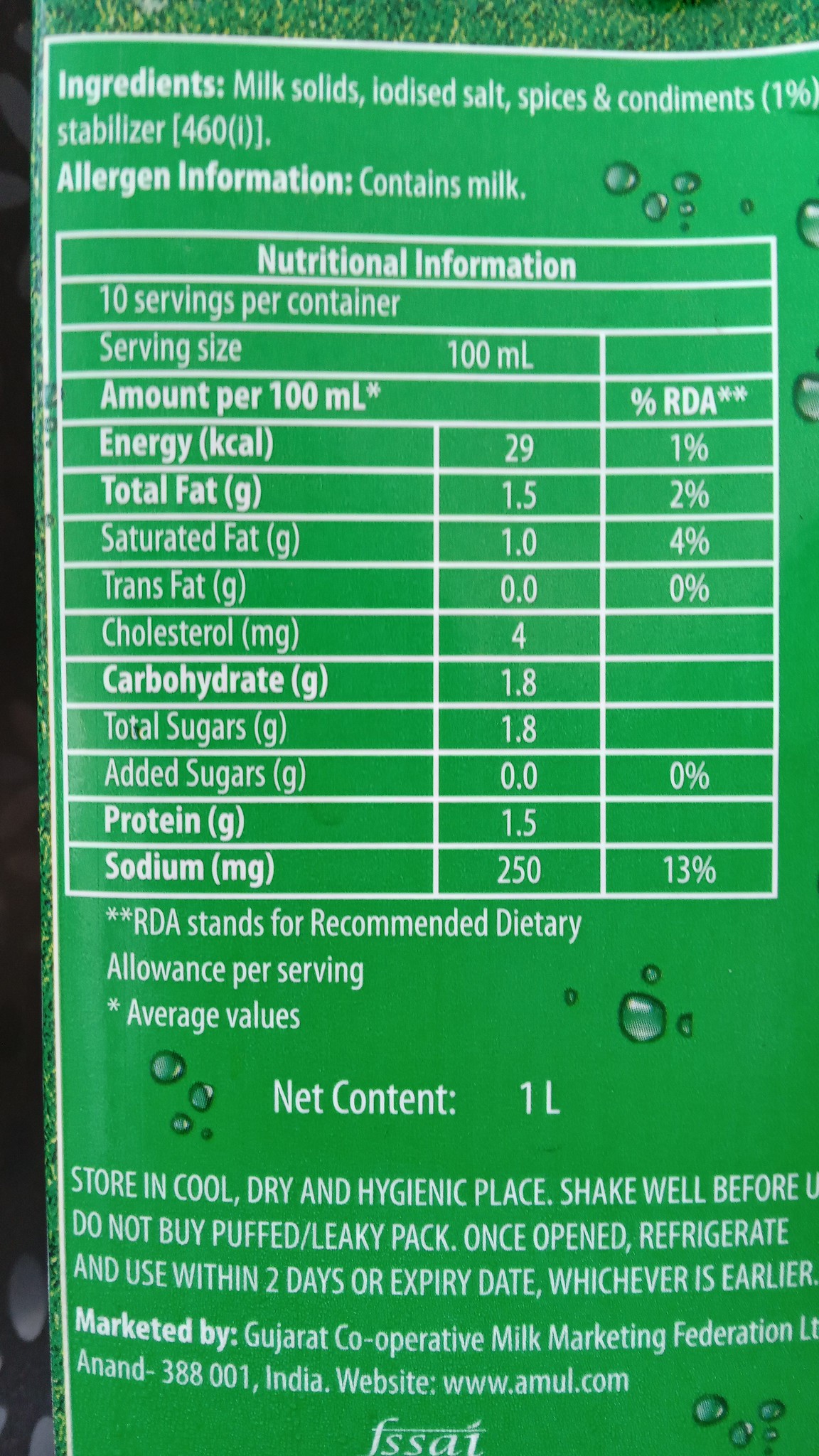This is a detailed color photograph of a rectangular product label that is taller than it is wide. The image is a close-up shot focusing on the back side of the product, specifically showcasing the nutritional information. The label features a green background with text organized in a structured manner. 

At the very top, the label lists the ingredients, prominently displaying items such as milk solids and iodized salt. Following this, there is a section with allergen information that explicitly states, "Choline contains milk."

Beneath the allergen information, a table is presented that details various nutritional values. This table includes information on serving size, energy, total fat, saturated fat, and other nutritional components, extending to just below the halfway point of the label.

Further down, the label includes additional nutritional information, such as Recommended Daily Allowance (RDA) percentages and average values, which provide context on the nutritional content. At the bottom of the label, the net content is specified as one liter. Below this, additional details are provided about storage instructions and the entity marketing the product. However, the photograph does not reveal enough information to clearly identify the product itself.